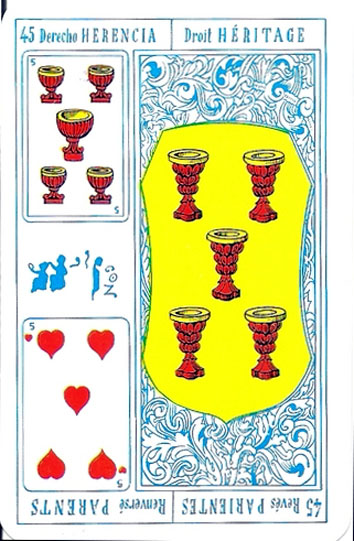The image depicts a vintage-inspired box of playing cards, displaying both Spanish and French text. The top section of the box shows "45 en derecho, herencia" in Spanish, and "Trois Héritage" in French. At the bottom left-hand corner, the text "45 Jueves Parientes" is written upside down, while the same text appears upright at the bottom right-hand corner.

The central illustration features a detailed, artistic representation reminiscent of 1800s style art. A blue rectangular box dominates the right side of the image, adorned with a white and blue pattern of intricate, curled leaves. Within this ornate frame is a yellow, curved shield shape, showcasing five red cups with gold interiors arranged in a suit-like pattern.

Additionally, at the bottom of the image, there is a depiction of a five of hearts card. The entire composition is bordered in blue, enhancing the antique aesthetic of the design. The vivid red and gold details of the cups accentuate the overall ornate and elaborate artistry of the playing card box.